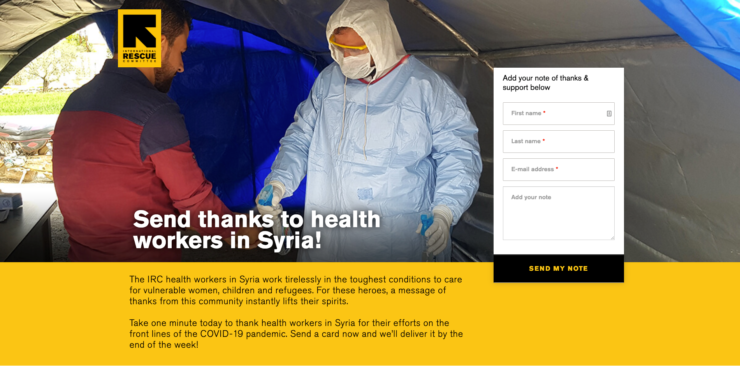In the image, we have a website titled "The Rescue," which prominently displays a large left-pointing arrow inside a yellow square. To the right of the arrow is the website's cover image, depicting an individual dressed in highly protective gear, resembling a hazmat suit. The person's face is partially obscured by protective goggles and a high-intensity face mask, with their head also covered. The suit they are wearing is blue. Positioned to the right of this image is a text prompt that reads, "Add your note of thanks and support below."

Beneath this text, there is a form contained within a white square. The form includes fields labeled "First Name," "Last Name," "Email Address," and "Phone." Below the form, there is a button with the text, "Send my note." Additionally, there is a call-to-action that says, "Send thanks to health workers in Syria." At the bottom of the image, there is a brief description in black text explaining the purpose of the website.